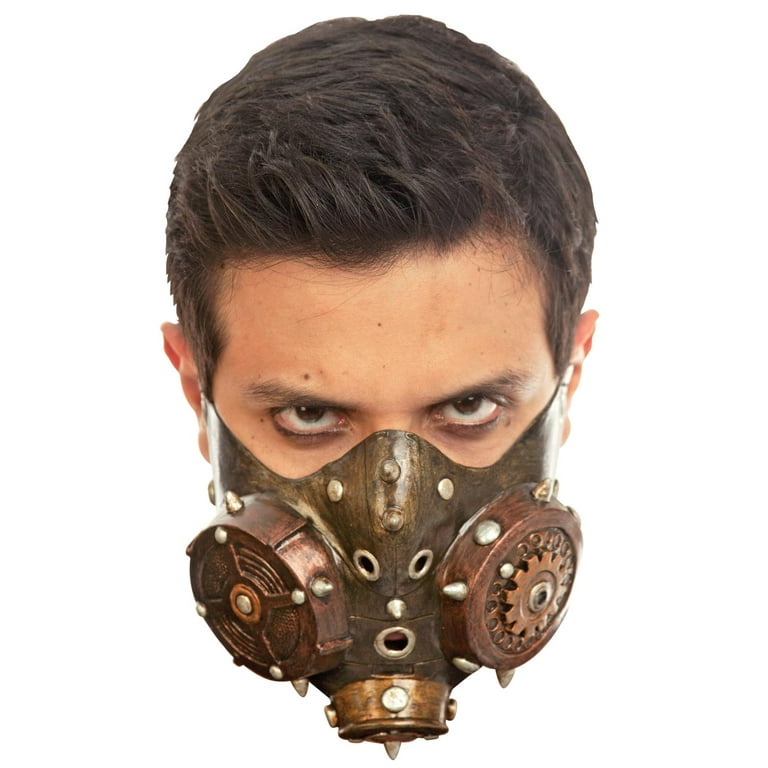The image depicts a man with dark brown, short hair styled upward in the front, extending to his ears and accompanied by sideburns. His piercing brown eyes are noticeably looking slightly upwards, directly at the camera. He is set against a plain white background. Prominently, he is wearing a distinctive steampunk-inspired gas mask that appears to be made of copper. The mask features a combination of dark and light copper hues, including studs and bolts giving it an intricate, industrial appearance. Notably, it has three circular filters or vents—one on each side and one at the bottom, with pairs of breathing holes and an array of round and pointy studs enhancing its aesthetic. The overall color scheme of the image includes tan, beige, brown, and copper tones. The mask secures behind his ears, suggestive of a pandemic-style design, but its elaborate detailing points towards a costume piece typical of the steampunk genre.